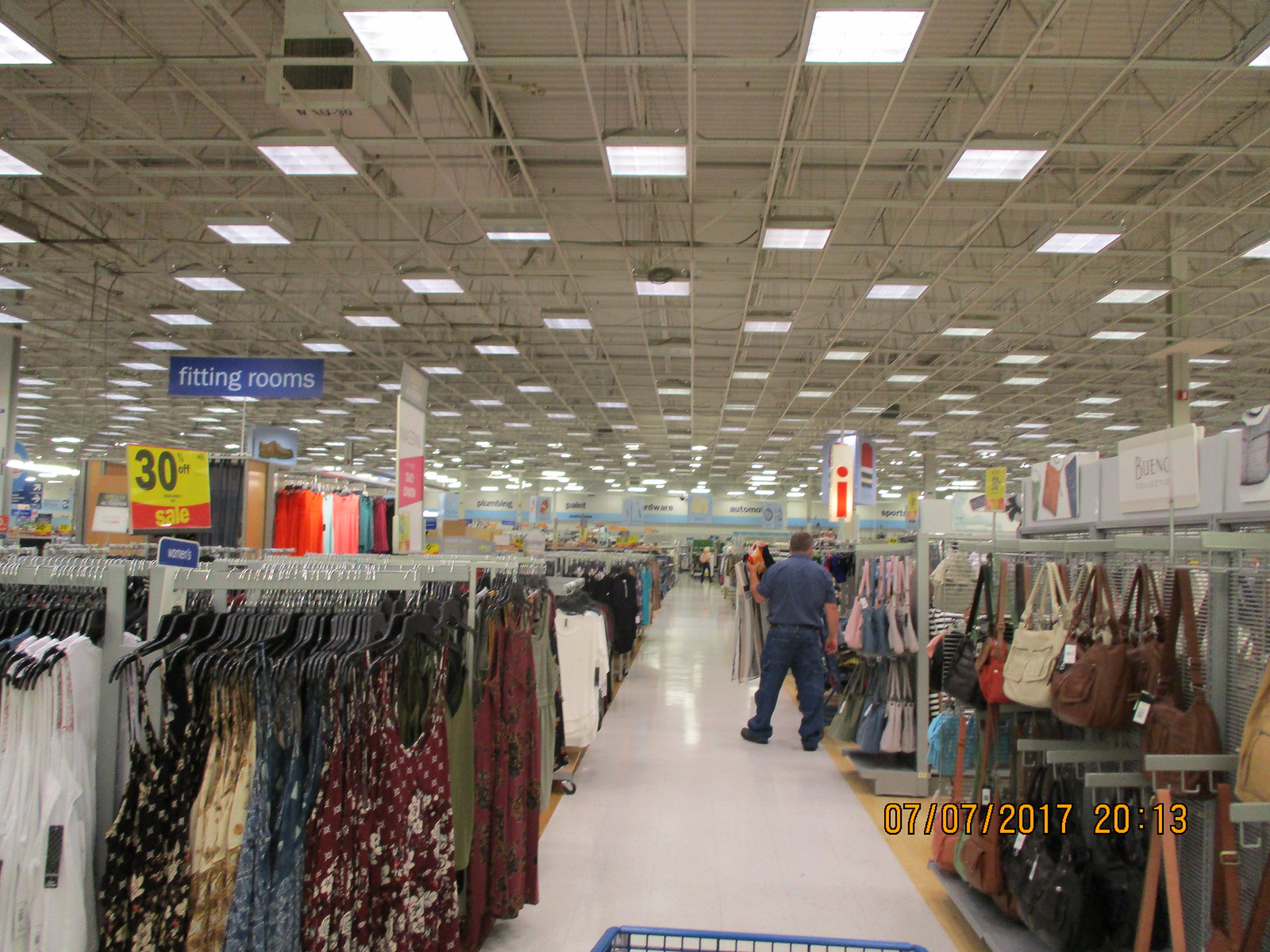The image captures an expansive department store, its vastness stretching nearly 100 meters down a single bustling aisle. This aisle is densely lined with racks of clothing, handbags, and various accessories, extending into numerous other areas brimming with merchandise. Standing centrally within the frame is a man dressed in a blue t-shirt and blue jeans, facing away from the camera. In the distant background, another individual is just visible at the far end of the aisle. The foreground subtly reveals the photographer’s shopping trolley, hinting at their position and movement. In the bottom right corner of the image, the timestamp "7th of the 7th 2017 2013" is noted. Overhead, a blue sign indicates the location of the fitting rooms. The ceiling is exposed, revealing an industrial setup with multiple lights but no tiles, giving a clear view of the building’s structural elements.